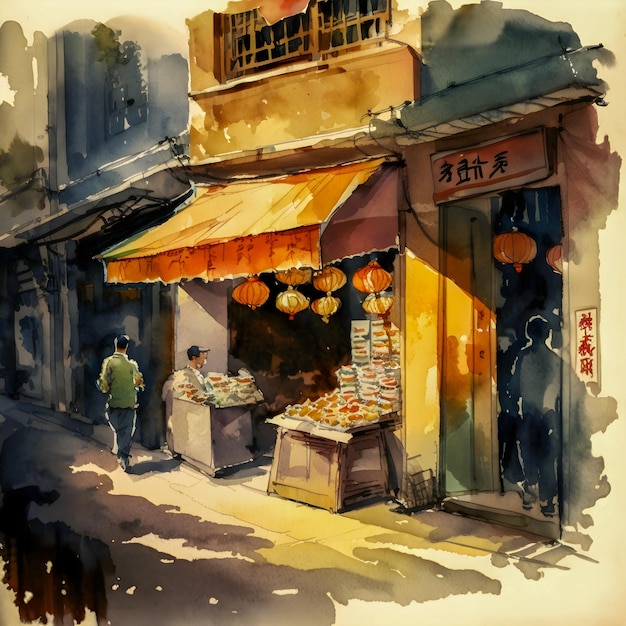This detailed watercolor painting, possibly digital but mimicking traditional watercolor, vividly captures a bustling street scene in an Asian city, likely Chinatown or an old-school Chinese neighborhood. Dominating the composition is an orange-brown storefront in the center, adorned with prominent Chinese characters on signs both above its entrance and on the right-hand side. The storefront features an orange-yellow awning with traditional red Asian lanterns hanging just underneath, casting a warm, inviting glow. Surrounding this central building, other structures can be seen—a blue building to the left and another blue building to the right.

The scene is lively and detailed, showcasing an array of products displayed on tables extending onto the street. The painting's warm tones are accentuated by deep shadows, especially on the left-hand side, highlighting the texture and color of the buildings. Three figures animate the scene: one person dressed in blue stands near the leftmost blue building, another appears to be a shopkeeper in the central building, identifiable by their baseball cap, and a third person is seen entering through an open door on the right, blending into the painting's gray and purple shadows. This richly detailed artwork encapsulates the essence of a vibrant, traditional Asian market street.